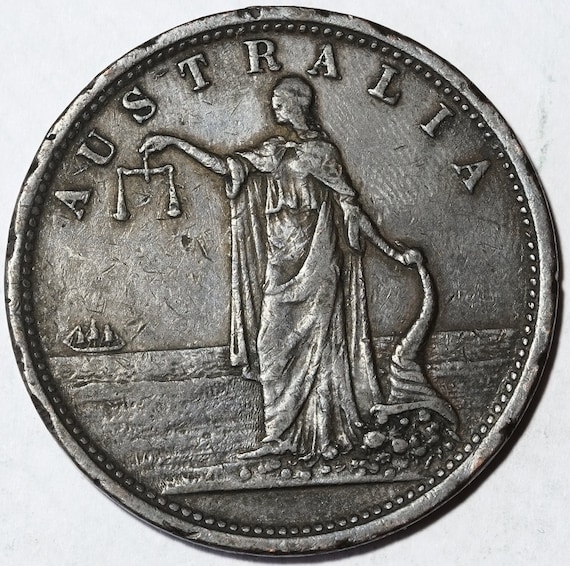This detailed close-up color photograph showcases an antique Australian coin with a silver metallic texture, occupying the entire image. Central to the coin is the engraved image of a woman standing before a sea, dressed in a long, flowing gown. She is holding balancing scales in one hand and a cornucopia or horn of plenty in the other, spilling its contents into the ocean. To the left of the woman, a ship with a couple of men sails away, adding to the coin's intricate design. The word "AUSTRALIA" is prominently displayed at the top in an old-fashioned, capitalized font. The overall impression is that of an aged, well-worn coin that has seen better days, set against a light gray or almost white background.